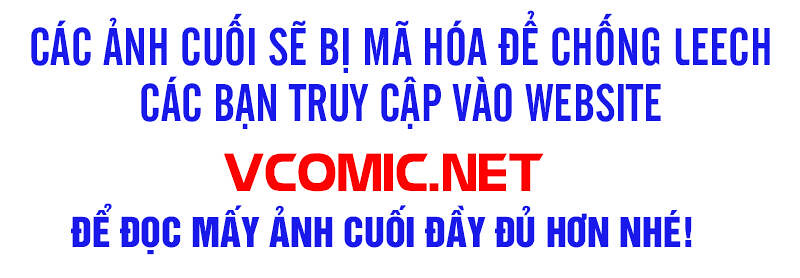The image features a plain white background with text in a foreign language that uses Latin letters, but it is certainly not in English. The text contains several accents on many of the vowels, suggesting it might be Vietnamese or from another Southeast Asian country. The primary text is in blue, likely serving an advertising purpose. Additionally, there is red text displaying the URL "vcomic.net".

Here is an attempt to transcribe the text phonetically based on an English speaker’s perspective: "sas-an-suo-se-bi-ma-hua-de-chong-li-ch. Sas-ban-trui-kap-vau-web-site. De-dok-mai-an-koi-dai-du-hon-ne." Though this transcription may not be accurate, it represents how an average American might read it.